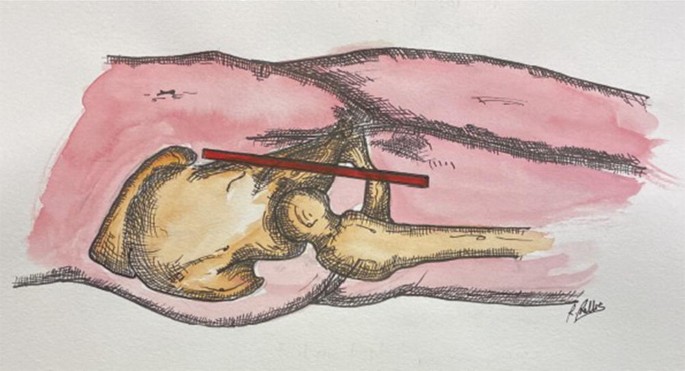The image is a detailed, abstract medical illustration, possibly a combination of chalk and ink with watercolor highlights. It depicts a horizontal view of a leg, focusing on the area from above the knee to a few inches below it. The leg's flesh is painted in red, while the bone inside is rendered in a light brown watercolor, adding depth and texture. A prominent red line runs straight through the knee joint, suggesting a medical intervention, maybe a fixation for a fracture. The muscles are depicted in pink, and the bones have a yellow tint with intricate shading. The overall composition hints at a professional diagram, similar to those found in medical textbooks or academic notebooks. A black signature is located in the bottom right corner, adding a final touch to this meticulous artwork.